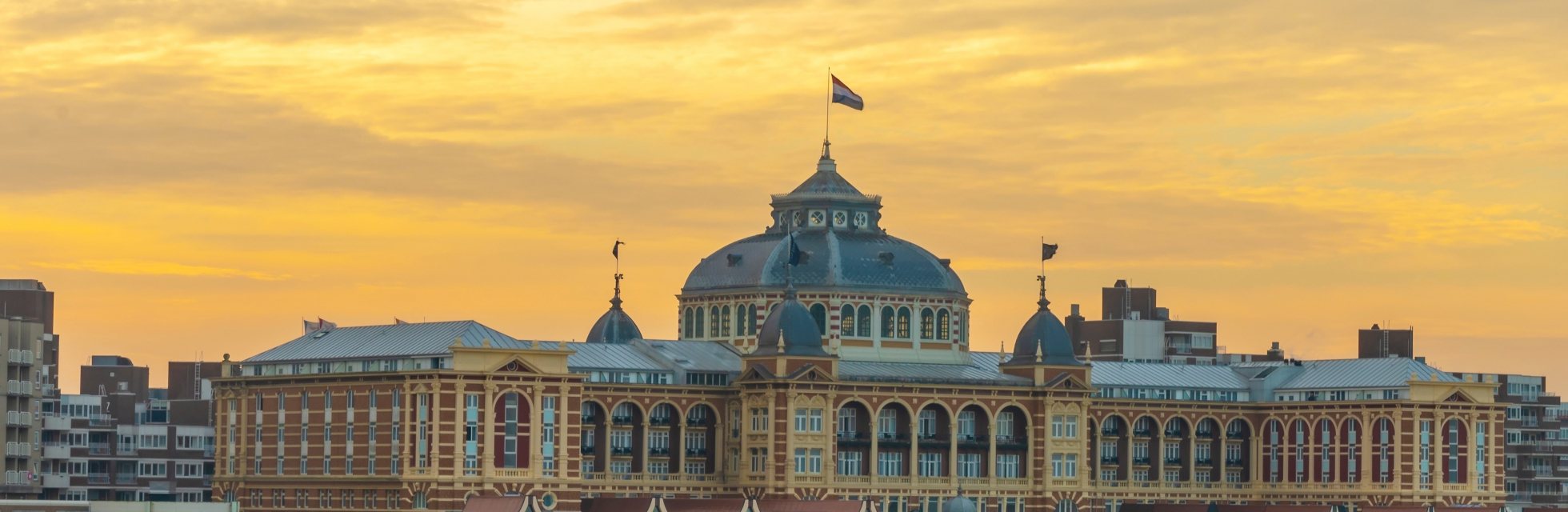This panoramic outdoor photograph captures a vast, impressive brick building that stretches across nearly the entire frame under a yellowish, sunset sky with reddish-brown clouds. This grand structure, possibly a large train station or government building, features a plethora of multi-story, arched windows with white trim and yellow brick highlights accenting its corners and columns. The building's red brick facade contrasts with its slate gray roof. At its center, a prominent, domed tower rises with a flag displaying vertical red, white, and blue stripes, flanked by two smaller domes each boasting their own flagpoles and flags. Behind the primary building, a cityscape with high-rise buildings can be glimpsed, adding depth to the scene. Despite being a detailed architectural marvel, no text or signage is visible in the image.